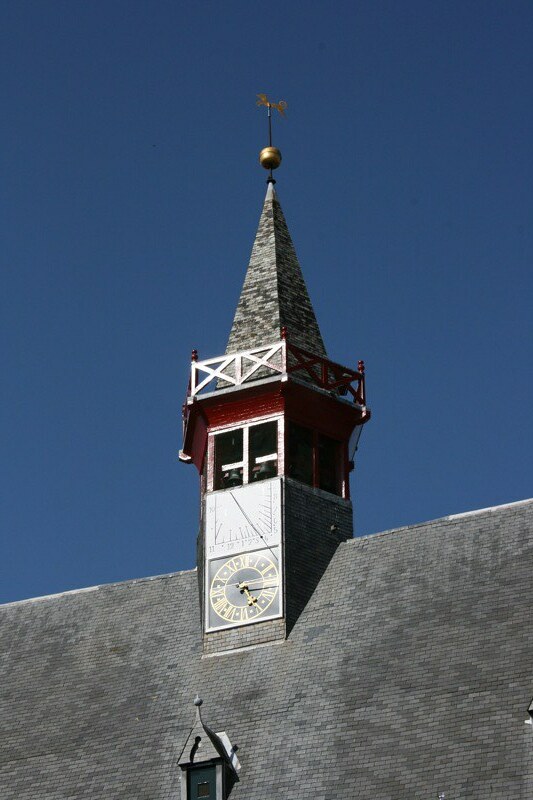In the image, an old Bavarian-German style building is prominently featured, showcasing its steeply sloped slate gray tiled roof. At the base of the roof, a small window with a dark green door peeks out, crowned by a tiny steeple-like structure. Above this, a grander steeple rises, adorned with a gilded brass figure of a dog perched atop a large, ornate bulb, also in brass or gold. The steeple culminates in a traditional spire, while at its base, a gilded clock displays the time as 5:10 PM. The vibrant blue sky accentuates the rich red brickwork that frames the clock, adding to the picturesque and historic charm of the building.